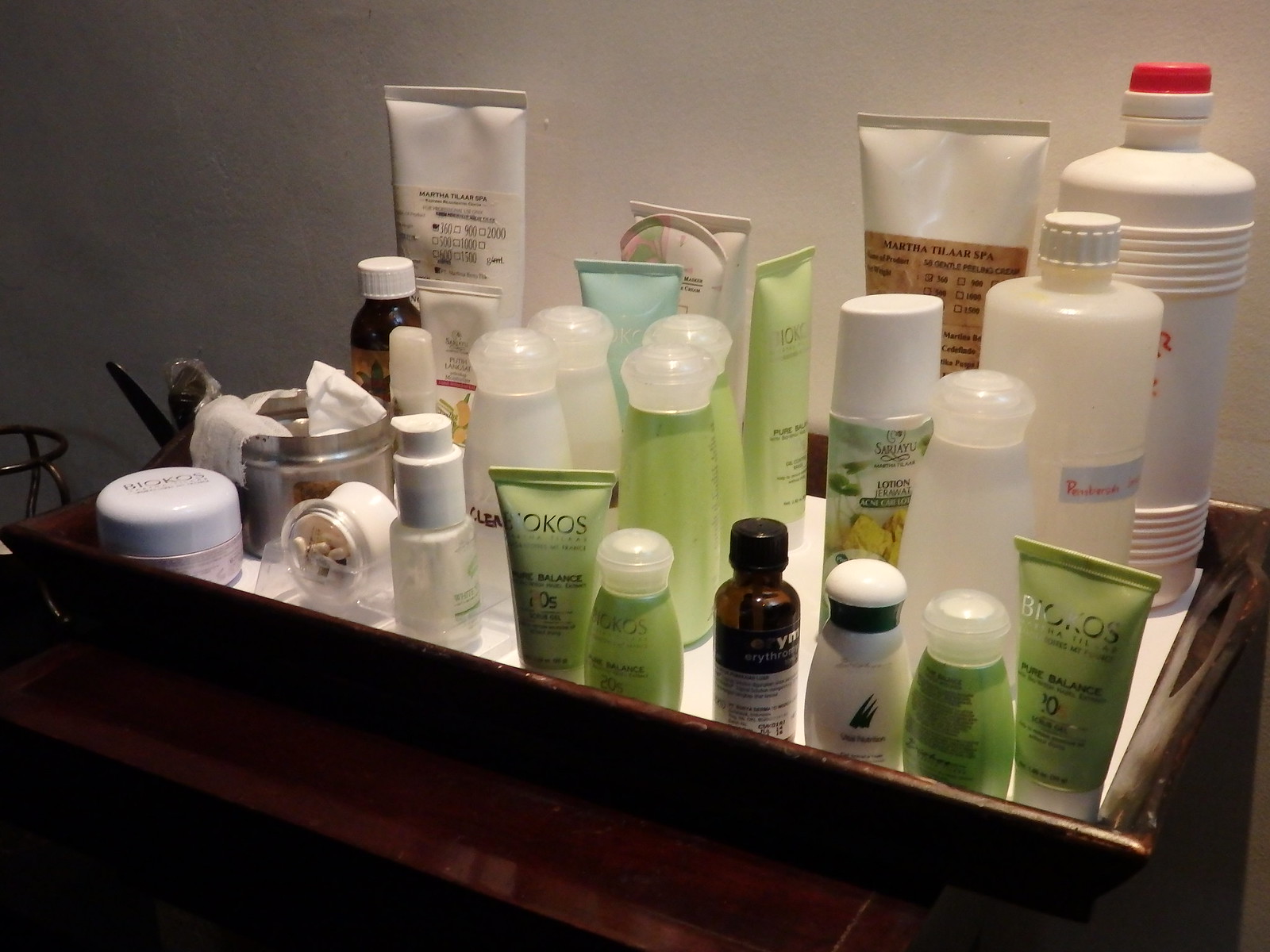In the image, a brown table is partially visible, primarily showing its top surface. Resting on the table is a brown tray that blends seamlessly with the table. The tray is filled with various cosmetic products, organized neatly. Among the products, there are several bottles and tubes. The tubes are of different colors, including green, white, and clear. Additionally, there are small brownish bottles, most of which have white lids. Notably, there is one bottle with a black lid, standing out among the otherwise uniform white lids. The diverse array of containers adds to the organized yet varied display of cosmetic products on the tray.